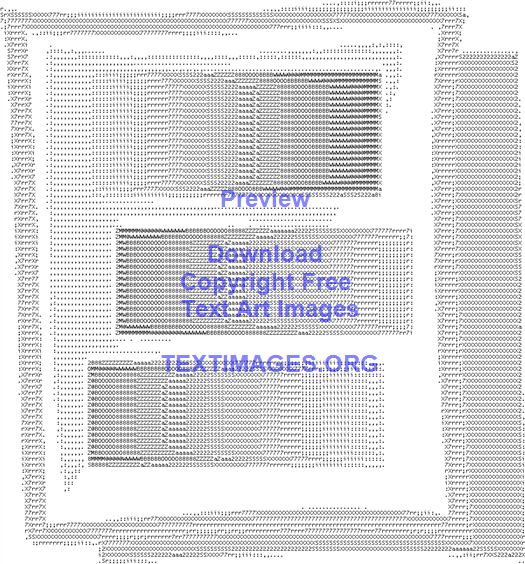The image displays a blurred, grayscale background that appears almost fabric-like, with various overlapping scratch-like markings that suggest an incomplete or corrupted download. Dominating the center, blue text reads "Preview," followed by "Download," "Copyright Free," "Text Art Images," and "Textimages.org" in all caps. The text is prominently displayed in a vertical list, with the rest of the image transitioning from light to dark gray, creating a faded effect across the background. The overall composition hints at a 3D object, possibly a pillow or fabric, though it's not entirely clear due to the blurriness and abstract nature of the image.